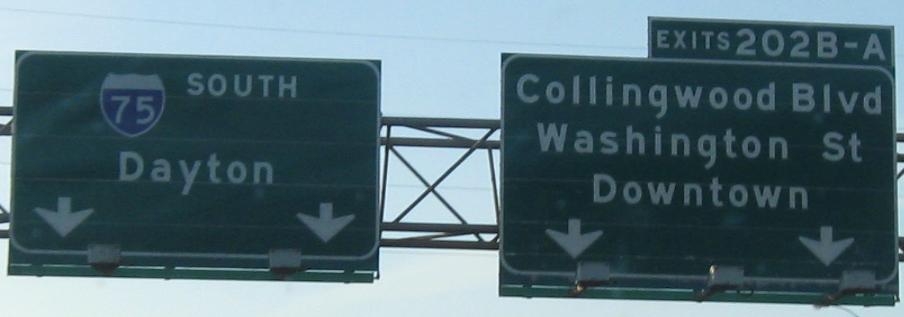This photograph captures two highway signs mounted on a metal scaffold, providing clear directions for drivers. Both signs are the standard green with white lettering common on highways.

The left sign directs traffic to "75 South Dayton," featuring two downward-pointing arrows indicating the lanes for this route. The right sign indicates "Exits 202B-A," with additional information pointing towards "Collingwood Boulevard," "Washington Street," and "Downtown." It also has two arrows pointing down to mark the specific lanes for these exits.

In the background, a cloudless blue sky suggests a bright, clear daytime setting. The signs appear slightly worn, hinting at years of service in guiding motorists.